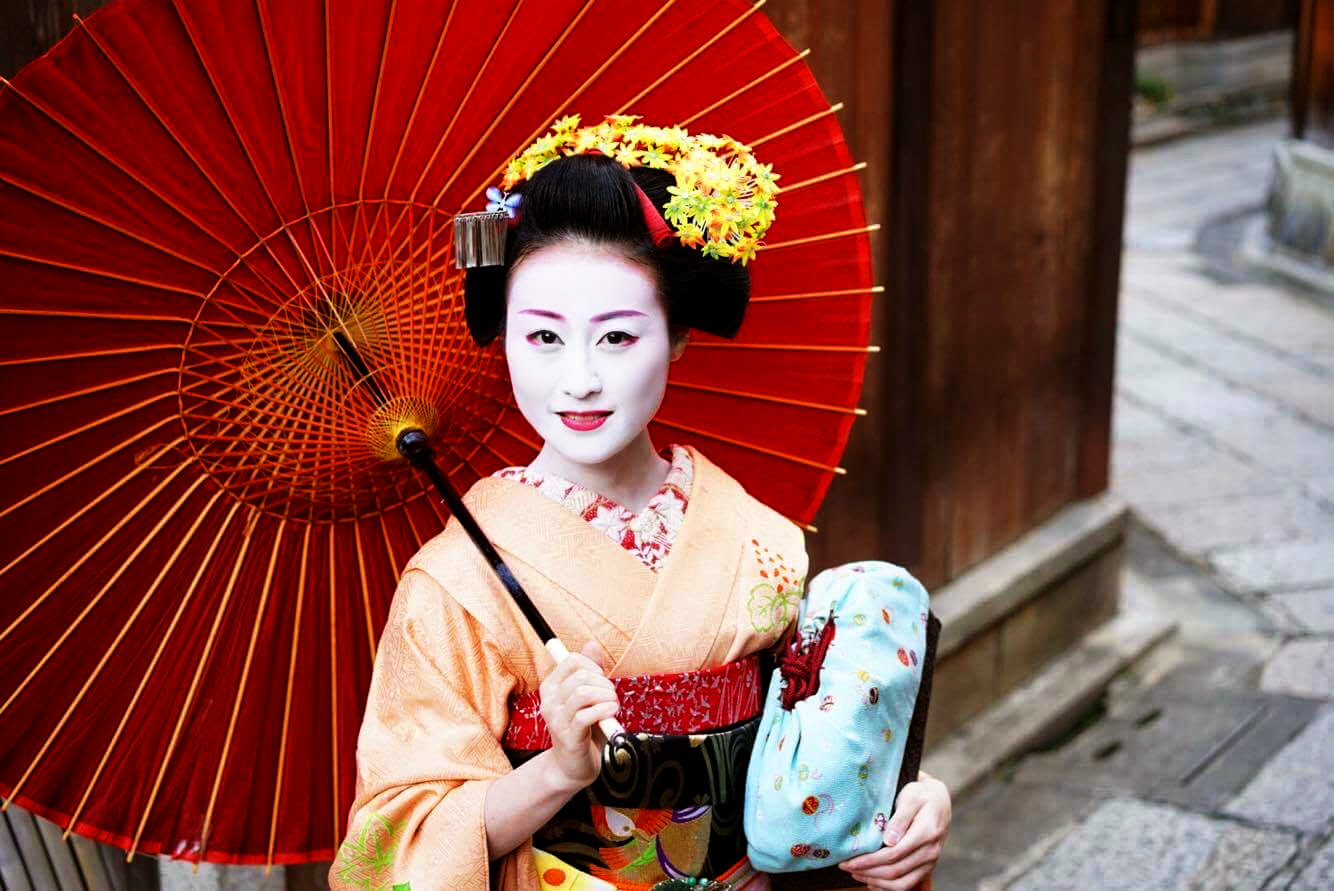The photograph depicts a Japanese woman, possibly a geisha, dressed in a traditional kimono. Her hair, intricately styled and pinned up, features a red hair band and yellow flowers arranged in a horseshoe shape, with some green and orange accents. Her face is covered with white makeup, and her lips are painted red, adding a delicate touch to her soft smile. She holds an open red umbrella with yellow accents in her right hand, which rests on her shoulder. Her kimono is primarily light orange or peach with a mix of white, red, green, and tan sections, and it is secured with both red and white belts. In her left hand, she carries a baby blue bag. She stands on a stone grey path that curves around, posed in front of a brown wooden building, adding a traditional backdrop to the scene.